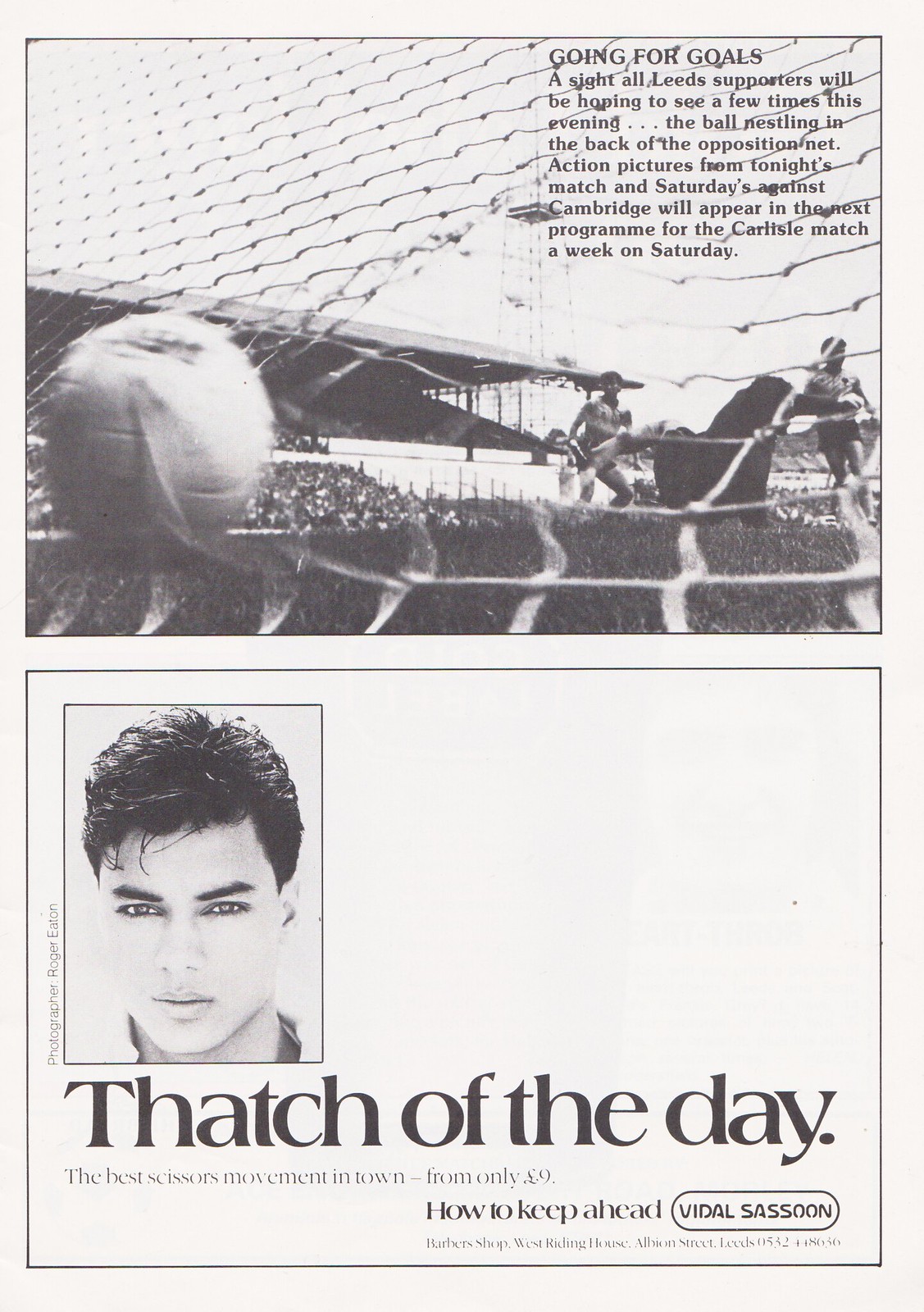This image is the front cover of a black and white game day program or magazine. The top half features a close-up photo from the backside of a soccer goal showcasing a ball hitting the net, positioned to the left. Overlaid on the image, towards the right, is a paragraph of text reading: "Going for Goals. A sight all Leeds supporters will be hoping to see a few times this evening. The ball nestling in the back of the opposition net. Action pictures from tonight's match and Saturday's against Cambridge will appear in the next program for the Carlisle match a week on Saturday." The bottom half of the page transitions into a blank white background with a portrait of a man with black hair staring neutrally to the left. Below his image, it states: "Thatch of the Day. The best scissors movement in town from only €9. How to keep ahead, Vidal Sassoon."